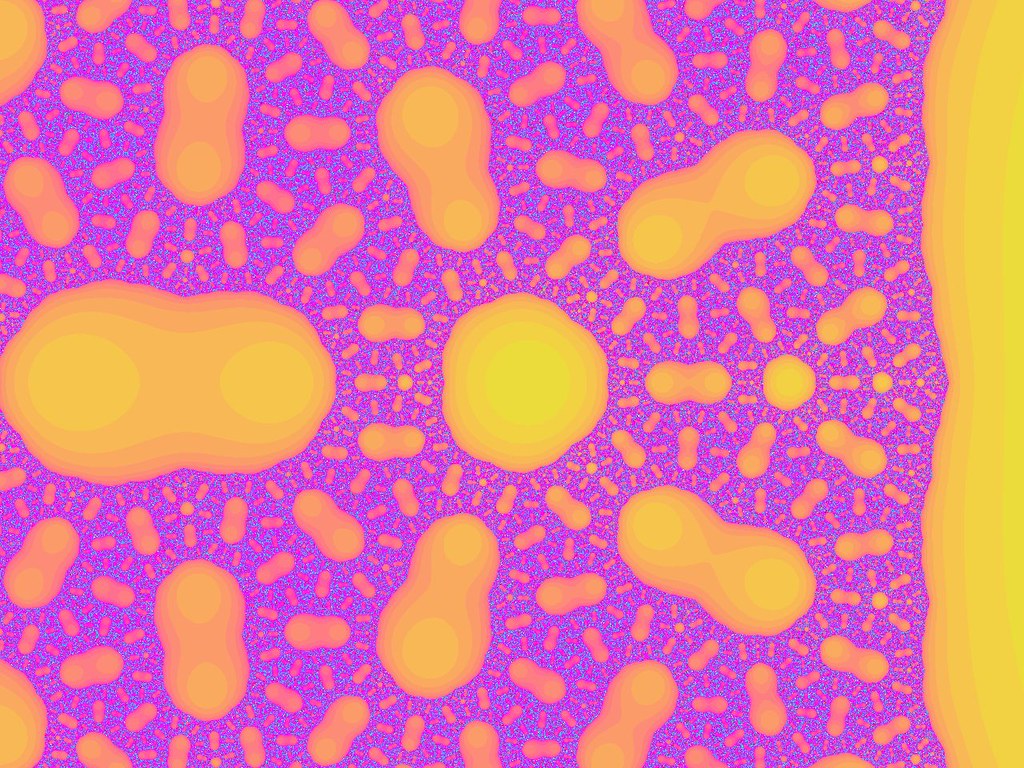This artwork features a vibrant purple background with various abstract shapes scattered throughout. The predominant shapes resemble peanuts in their shells, rendered in a gradient of yellow to orange and lined with deeper orange around the edges. These peanut-like forms vary in size, from tiny specks to significantly larger, irregularly round shapes that almost occupy the entire composition. The overall effect is dynamic, with the yellow and orange shapes seemingly floating or flying across the bright purple backdrop, creating a sense of movement and energy.